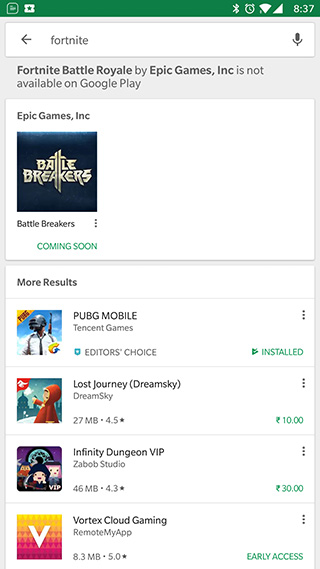This image is a detailed screenshot of the Google Play Store showcasing a search query for "fortnite." At the top of the screenshot is the Google Play Store search bar with "fortnite" typed in lowercase letters. To the left of the text within the search bar is a back arrow icon, and to the right is a microphone icon for voice search options.

Directly below the search bar, the text clearly states, "Fortnite Battle Royale by Epic Games Inc. is not available on Google Play." Beneath this message is a prominent white box highlighting another game by Epic Games titled "Battle Breakers." Accompanying this title is a square thumbnail image representing the game. Towards the bottom left corner of this section, the phrase "Coming Soon" is displayed in blue text.

Following the game advertisement, the screenshot shows the "More Results" section, presenting a vertical list of alternative games. The visible titles are "PUBG Mobile," "Lost Journey," "Infinity Dungeon VIP," and "Vortex Cloud Gaming." The rest of the page content isn't visible, as the screenshot is cropped.